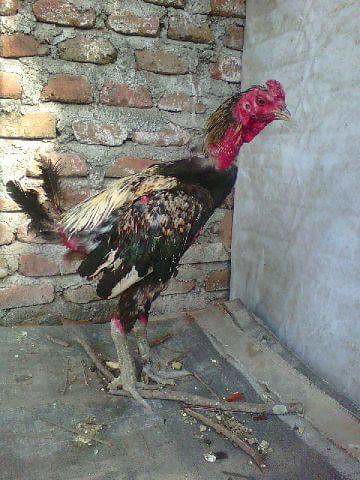The image captures an outdoor scene featuring an aged rooster standing on a concrete ground littered with sticks and debris. The rooster, characterized by a red face and a gray beak, displays a mix of tan, green, brown, black, white, and red feathers, although it appears to have lost many feathers near its tail and neck. Its legs are long and thick, with a grayish or tan coloration. The background consists of a red and brown brick wall, possibly the side of a house, with a substantial amount of visible mortar. The photograph is grainy, adding to the sense of wear and age both in the rooster and the setting.